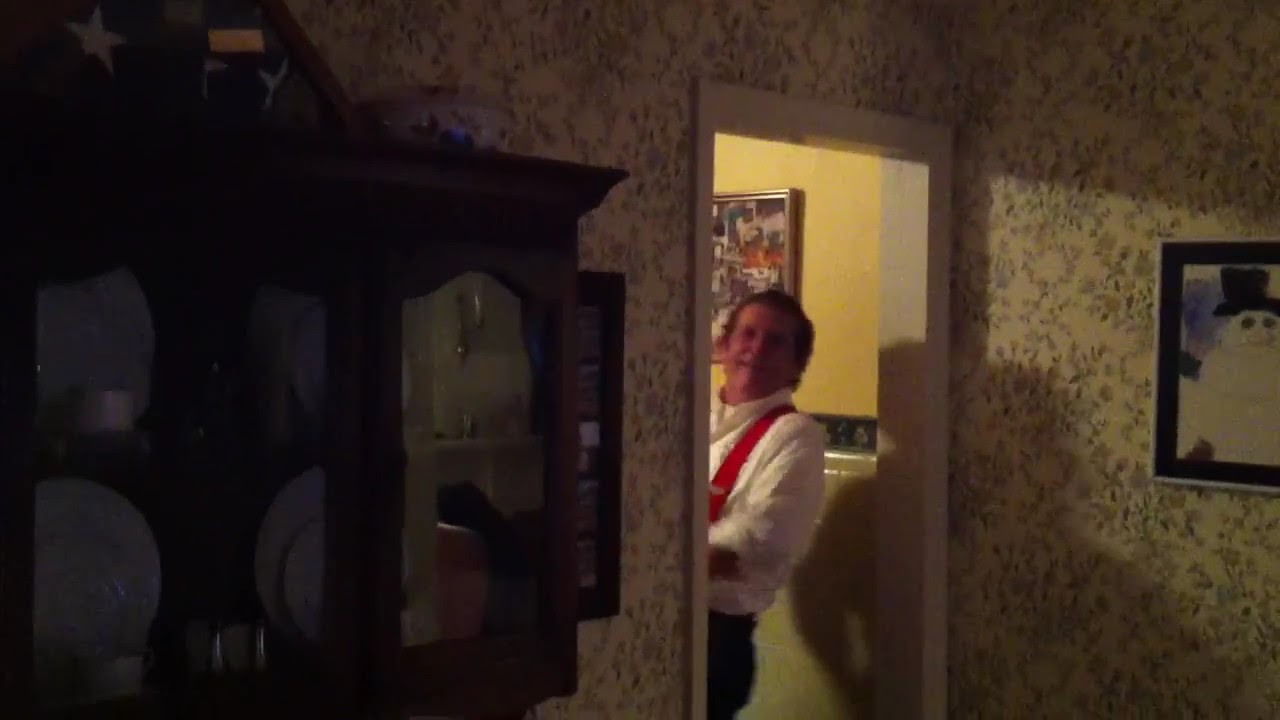The image depicts the interior of an older home, characterized by its vintage yellow wallpaper adorned with a busy floral pattern. The room is dimly lit, with the primary light source coming from a doorway that reveals a man standing just beyond the threshold. The man, with short brown hair, is wearing a white button-down shirt with the sleeves rolled up and bright red suspenders. He appears to be smiling or speaking while peeking through the doorway. To the left of the doorway, inside the room, stands a wooden armoire with multiple glass panels showcasing fine china. On the right side of the doorway, a framed picture of a snowman adds a whimsical touch. In the adjoining room, partially visible, is a washing machine, further emphasizing the charming, lived-in feel of the home.